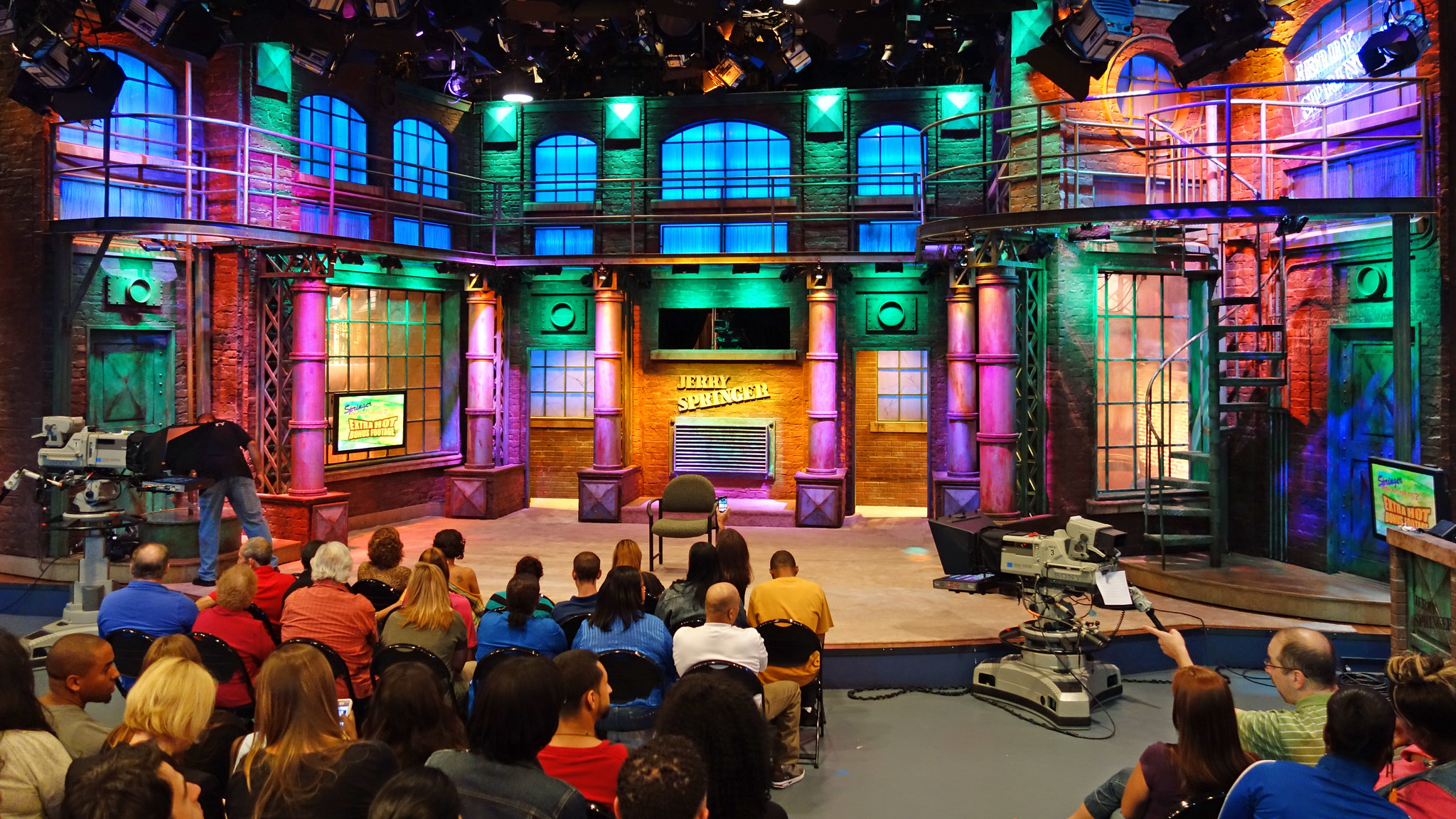The image depicts the bustling set of the Jerry Springer show, clearly identified by the text "Jerry Springer" along the back wall. The set is housed in a brick building adorned with windows, columns, and doorways. The stage occupies the center, featuring a single chair and is illuminated by a blend of green, purple, and warm white lighting. Above, a walkway and a spiral staircase on the right provide access to an upper level. Spotlights are mounted on metal racks across the ceiling, enhancing the set's visibility.

In the audience area, viewers are seated in folding black metal chairs, their backs turned to the camera. Large studio cameras, some light gray and on wheels, are strategically positioned between the audience and the stage, ready to capture the action. At the bottom left and right of the image, more audience members can be seen, one of whom is pointing towards the stage. On the stage, a man dressed in a black shirt and blue jeans is leaning forward, seemingly adjusting part of the set. The entire scene is framed with a sense of anticipation, capturing the lively atmosphere of the television show.